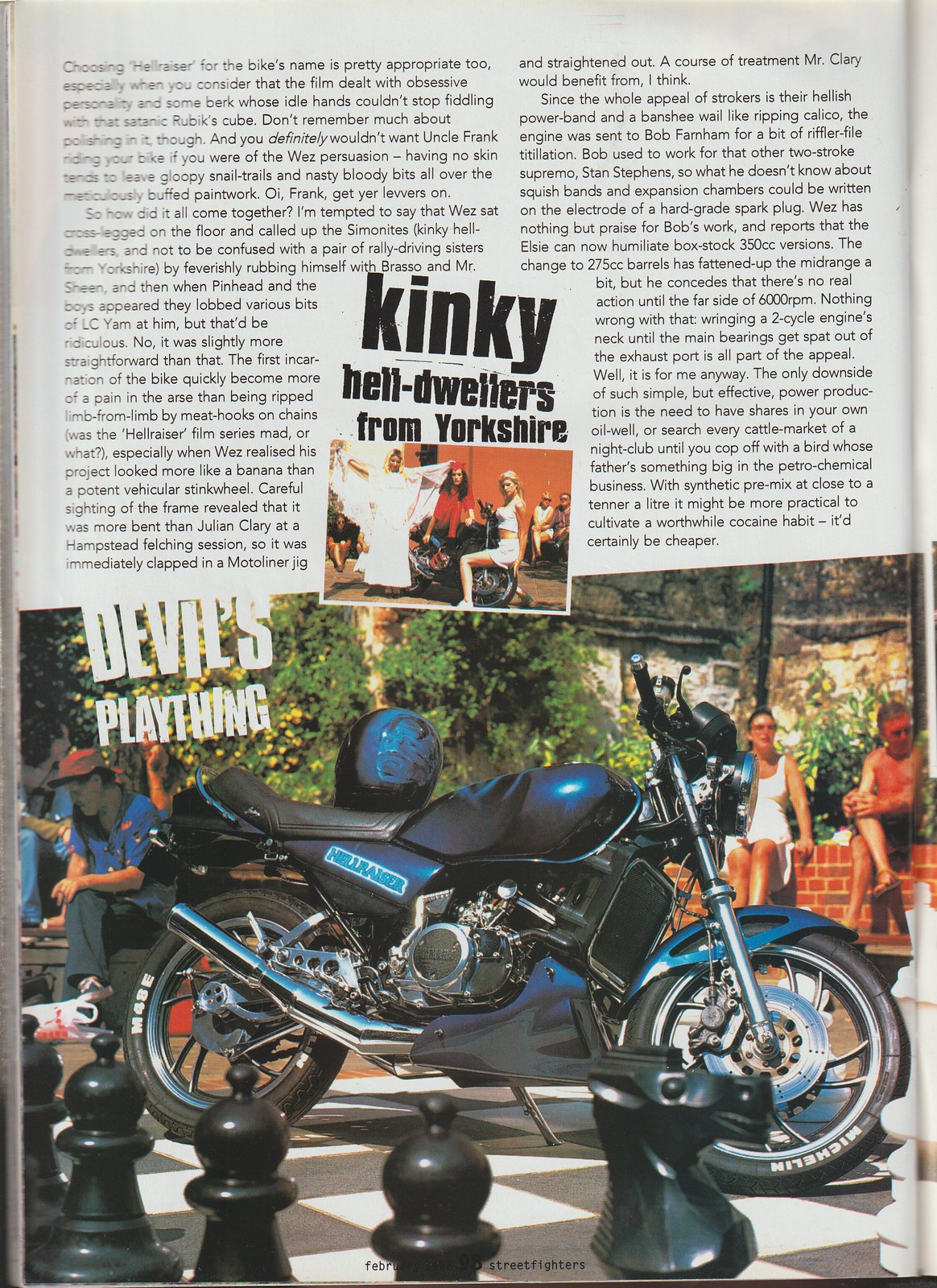The image is a detailed depiction from a magazine page, split into two halves. The upper half contains a black-and-white article with bold text proclaiming "Kinky Hell Dwellers from Yorkshire," accompanied by a small image of women posing on a motorcycle. The lower half of the page prominently features a photograph of a striking blue motorcycle with black seats and chrome detailing, including a blue-trimmed helmet. The motorcycle stands on a black-and-white checkerboard floor, resembling a large chessboard with oversized chess pieces scattered around. Bold white text near the motorcycle reads "Devil's Plaything." In the background, people can be seen sitting and standing, with trees indicating the outdoor setting.